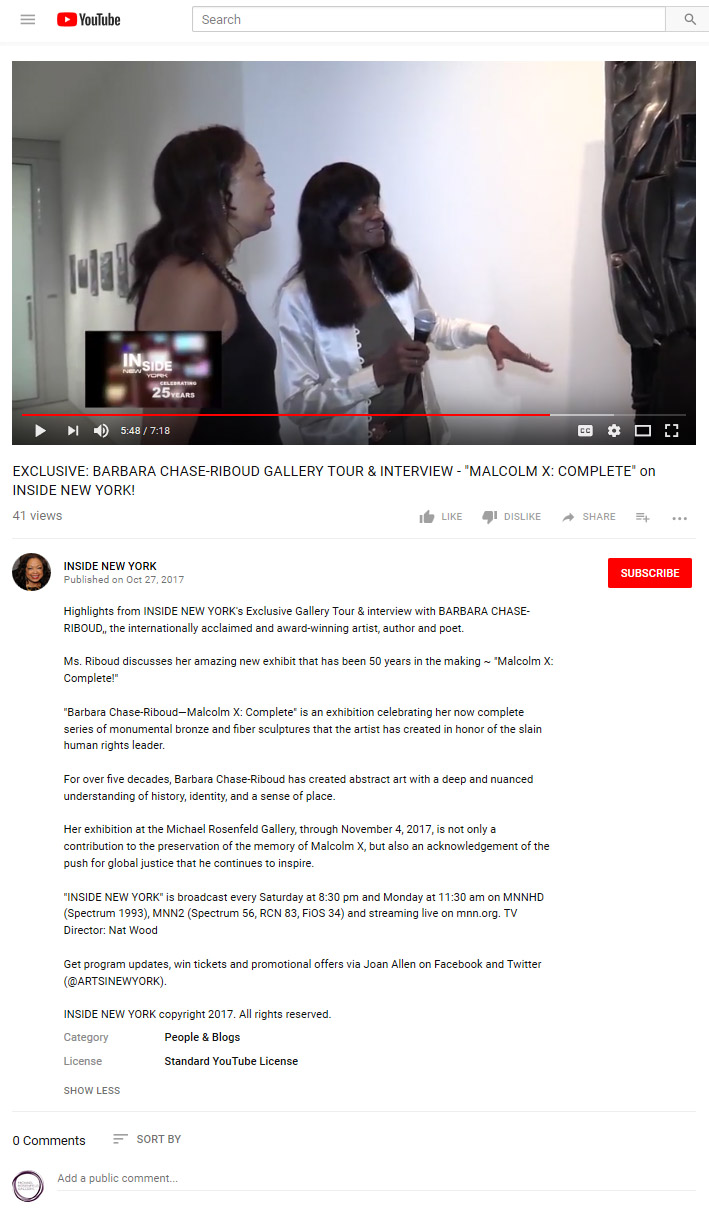This image is a screenshot of a YouTube video featuring the familiar white background of the platform. Along the top, the YouTube logo and a search bar are prominently displayed. Directly below this, an image captures a paused video at the timestamp of 5 minutes and 48 seconds into its 17 minutes and 18 seconds length. The paused frame shows two women standing next to each other against a white wall.

The video's title, "Exclusive Barbara Chase Reibold Gallery Tour and Interview | Malcolm X Complete | Inside New York," is displayed prominently. It has garnered 41 views. Below the video, there's a description from the uploader, Inside New York, indicating that the video was published on October 27, 2017.

The description provides highlights from Inside New York's exclusive gallery tour and interview with Barbara Chase Reibold, a renowned author, artist, and poet. In the interview, Reibold discusses her impressive new exhibit, "Malcolm X Complete," which has been 50 years in the making. The exhibition celebrates her finalized series of monumental bronze and fiber sculptures dedicated to Malcolm X, the iconic human rights leader.

For over five decades, Barbara Chase Reibold has been creating abstract art that embodies a profound understanding of history, identity, and a sense of place. Her exhibition at the Michael Rosenfield Gallery, running through November 4, 2017, not only honors the legacy of Malcolm X but also recognizes his ongoing influence in the quest for global justice.

The description also notes that Inside New York is broadcast every Saturday at 8:30 p.m. and Monday at 11:30 a.m. on MNHD Spectrum 1993, MNN2 Spectrum 56, RCN 83, Fios 34, and streams live on MNM.org.